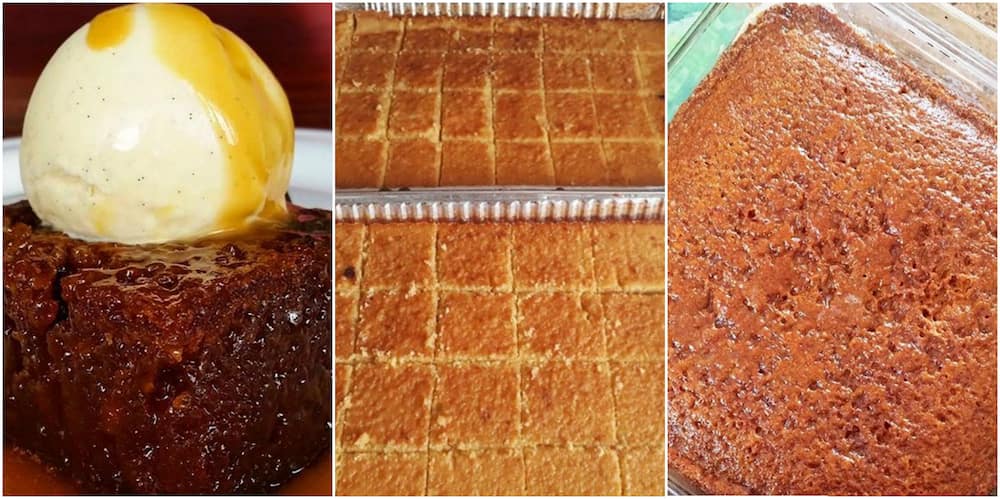The image showcases a series of three vertical, side-by-side photographs of various desserts. On the far left, there's a close-cropped shot of a glossy, dark rectangular cake, which appears to be a sticky toffee pudding adorned with a perfectly spherical scoop of vanilla bean ice cream and a caramel drizzle seeping underneath on a white plate. The middle photo captures a sheet cake or cornbread with a golden-brown top, already cut into neat squares still nestled within their baking pans, forming a grid-like pattern. The far right image features an overhead view of a square, golden-brown cake in a glass Pyrex dish, oriented diagonally within the frame. The images highlight a delightful assortment of cakes in different presentations, emphasizing textures, colors, and delectable toppings.